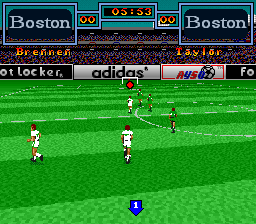Screenshot of a vintage 8 or 16-bit video game capturing an intense soccer match. The scoreboard displays "Boston" for both competing teams, with individual player names "Brennan" and "Taylor" listed under each. The match is a stalemate, both teams holding at zero points, with 5 minutes and 53 seconds remaining on the game clock. On the sidelines, vibrant banners featuring "Foot Locker," "Adidas," and "ASAO2" add a touch of realism to the retro aesthetic. The field hosts animated, pixelated players with brown skin and hair, donned in white and green, or green and black uniforms, energetically competing for control of the ball.